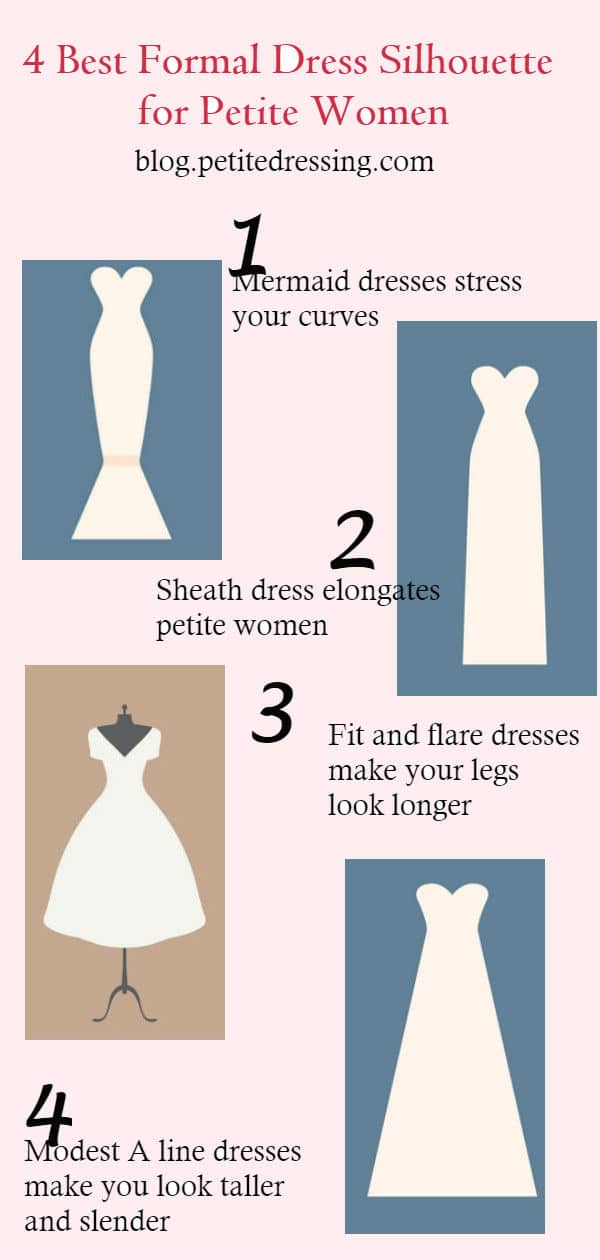The image is a digital, portrait-oriented, color illustration designed as an informational graphic likely meant for a website. The background is light pink with a headline at the top in red text that reads, "Four Best Formal Dress Silhouettes for Petite Women." Below the headline, in black text, it says, "blog.petitedressing.com." The graphic features four vertically-aligned panels, each illustrating a different dress type suited for petite women.

1. The first panel at the top left has a teal blue background with the illustration of a white strapless mermaid dress. This dress is tight-fitting to the knees and then flares out dramatically. The accompanying text reads, "Mermaid Dress Stresses Your Curves."

2. The second panel on the top right, against a teal background, displays a white sheath dress, which is straight and slim without any curves. The text beside it states, "Sheath Dress Elongates Petite Women."

3. The third panel, beneath the first, on a beige background, showcases a fit-and-flare cocktail dress on a mannequin. This dress is fitted at the top and flares out into a triangle shape towards the bottom. The text highlights, "Fit and Flare Dresses Make Your Legs Look Longer."

4. The fourth panel, positioned at the bottom right with a teal background, shows another long, white dress but this time appearing strapless and with a slight flare. The text beside it reads, "Modest A-Line Dresses Make You Look Taller and Slender."

The graphic design employs a harmonious color scheme with red, pink, blue, beige, black, and white, and combines typography with stylized dress illustrations. While the objects are well-positioned, there's slight overlap, adding to the layered, graphical layout. The overall style is clean, professional, and visually engaging, serving as both an advertisement and informative guide for petite women's formal dress choices.